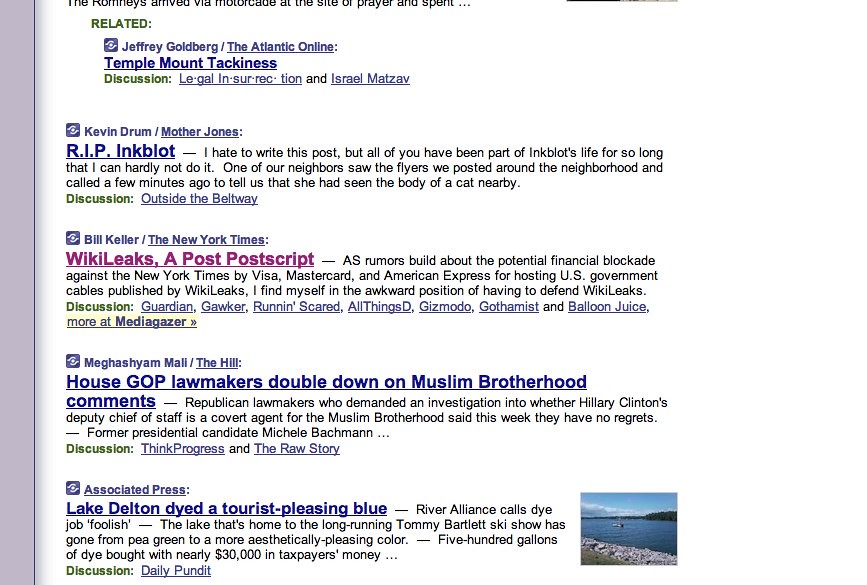The image features a screen displaying an organized collection of headlines and discussions from various publishers, emphasizing different topics. At the top, the word "related" appears in green. Below this is an underlined mention of "Jeffrey Goldberg — The Atlantic Online" with the title "Temple Mount Tackiness" in blue and underlined. 

Following this, the word "discussion" is highlighted in green. The next segment introduces "Kevin Drum — Mother Jones," with a bolder blue title "RIP Inkblot," followed by three sentences expanding on the topic. Below this, "discussion" appears once more in green, and "Outside the Beltway" is underlined.

Further down, "Bill Keller — The New York Times" is mentioned, under which is a purple title "WikiLeaks, a Post Postscript." The subsequent category lists "Megan Scheinman Male — The Hill," followed by a bolder blue headline "House GOP Lawmakers Double Down on Muslim Brotherhood Comments."

The final category is from the "Associated Press," underlined, followed by a blue headline "Lake Delton Dyed a Tourist-Pleasing Blue." To the right, the image displays a picturesque view of blue water with mountains in the background, rocks, and some grass near the left corner adjacent to the water.